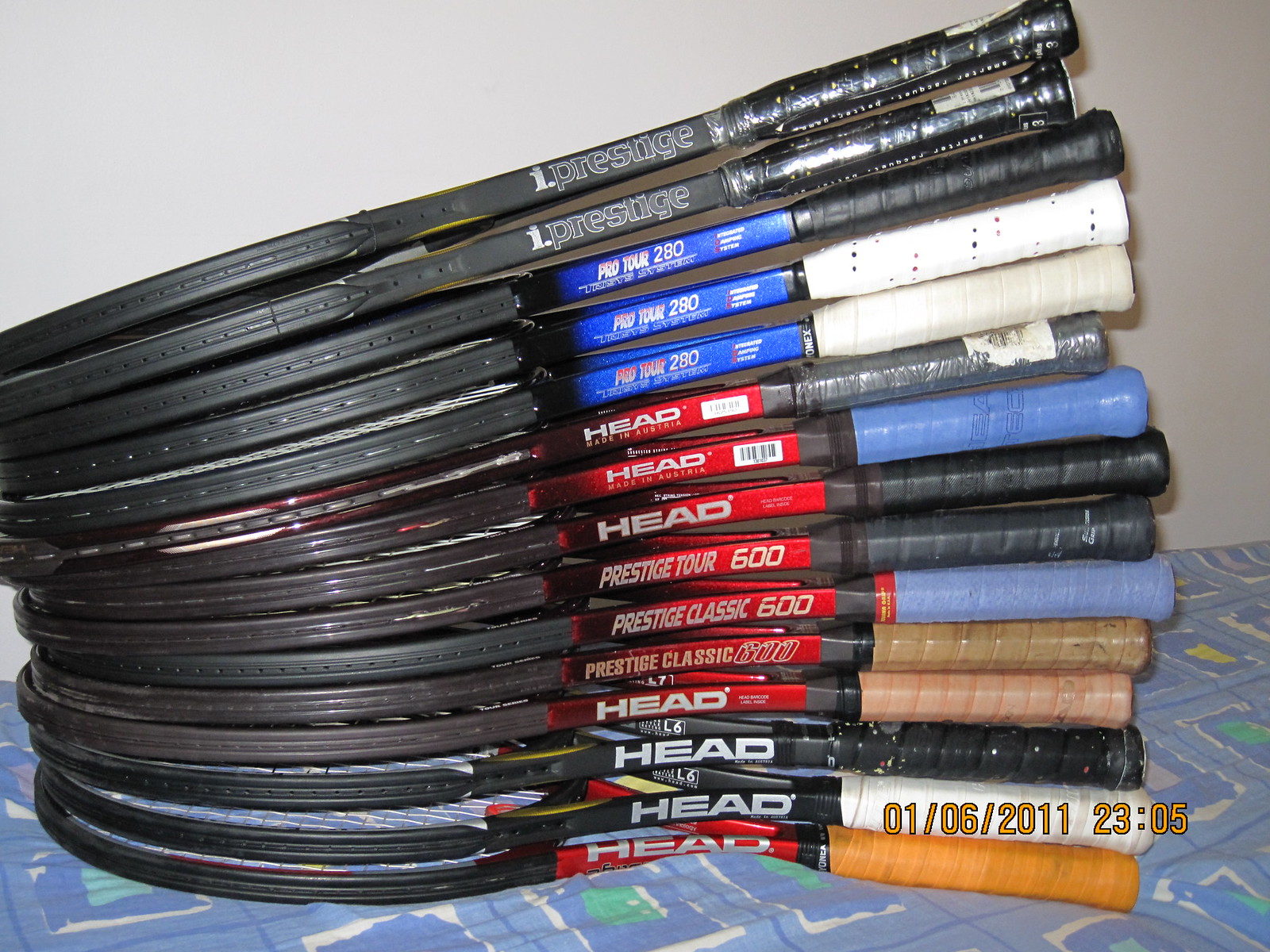The image features a meticulously stacked collection of tennis rackets viewed from a side profile, revealing their black frames, handle colors, and brand labels. The rackets, arranged with their heads on the left and handles on the right, showcase a variety of colors: the top three handles are black, followed by two white, one black, one blue, two more black, another blue, two brown, another black, one white, and one yellow handle. Notably, the rackets display a range of brand names such as iPrestige, Pro Tour 280, Prestige Tour 600, Prestige Classic 600, and numerous Head logos. The stack sits on a blue patterned fabric featuring blue squares with yellow and green details, set against a white wall in the background. A timestamp watermark at the bottom right corner reads "01-06-2011 at 23:05," indicating the photo was taken on January 6, 2011, at 11:05 PM.